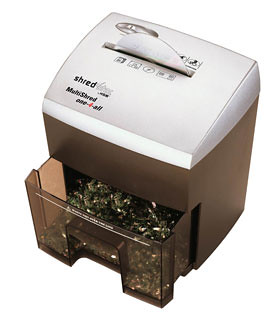The image reveals a meticulously presented shredder, photographed from a high, 45-degree angle against a stark white background. The shredder, appearing either photoshopped or crisply cut out, displays a combination of materials and colors. The top of the shredder is predominantly a silvery white plastic with a specific slot designed for shredding CDs and possibly other media, as evidenced by the half-inserted compact disc. The word "shred" and the phrase "multi-shred" are printed in black on the bottom left of the top surface. A toggle type switch, oval in shape, is situated in the top left corner, suggesting it serves as the power control. The sides and front of the shredder beneath the top appear to be constructed from a black plastic material, transitioning into a bronzy brown translucent drawer that is slightly pulled out. Through this drawer, we can glimpse the shredded remains of CDs, indicating the shredder’s capability to handle multimedia items. An indented handle in the middle of the drawer facilitates easy removal for emptying the contents. Overall, the shredder seems compact and suitable for personal or small office use, designed to sit on a desk or floor, effectively managing mixed media shredding tasks.